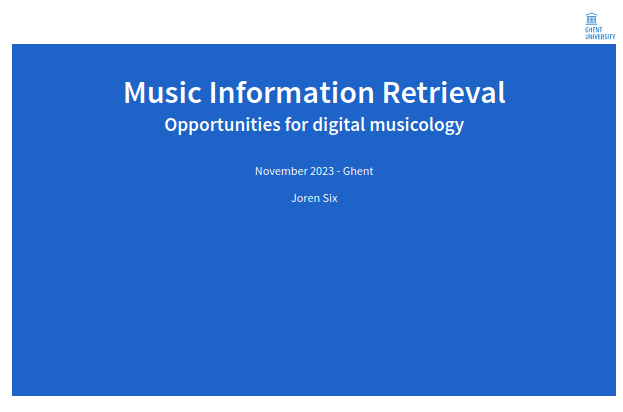The image features a rectangular, dark royal blue background, resembling a computer screen. Positioned at the top, there's an insignia of a three-arched building with a slanted roof, accompanied by the barely discernible name, "Ghent University," in very small lettering. Centered on the upper half of the background, prominent white bold letters spell out "Music Information Retrieval." Directly beneath this, in slightly smaller but still white font, the text reads "Opportunities for Digital Musicology." Below that, in even smaller white text, it states "November 2023, Ghent." The final line of text, also in small white letters, says "Jorin 6." The lower half of the blue background remains plain and unadorned.